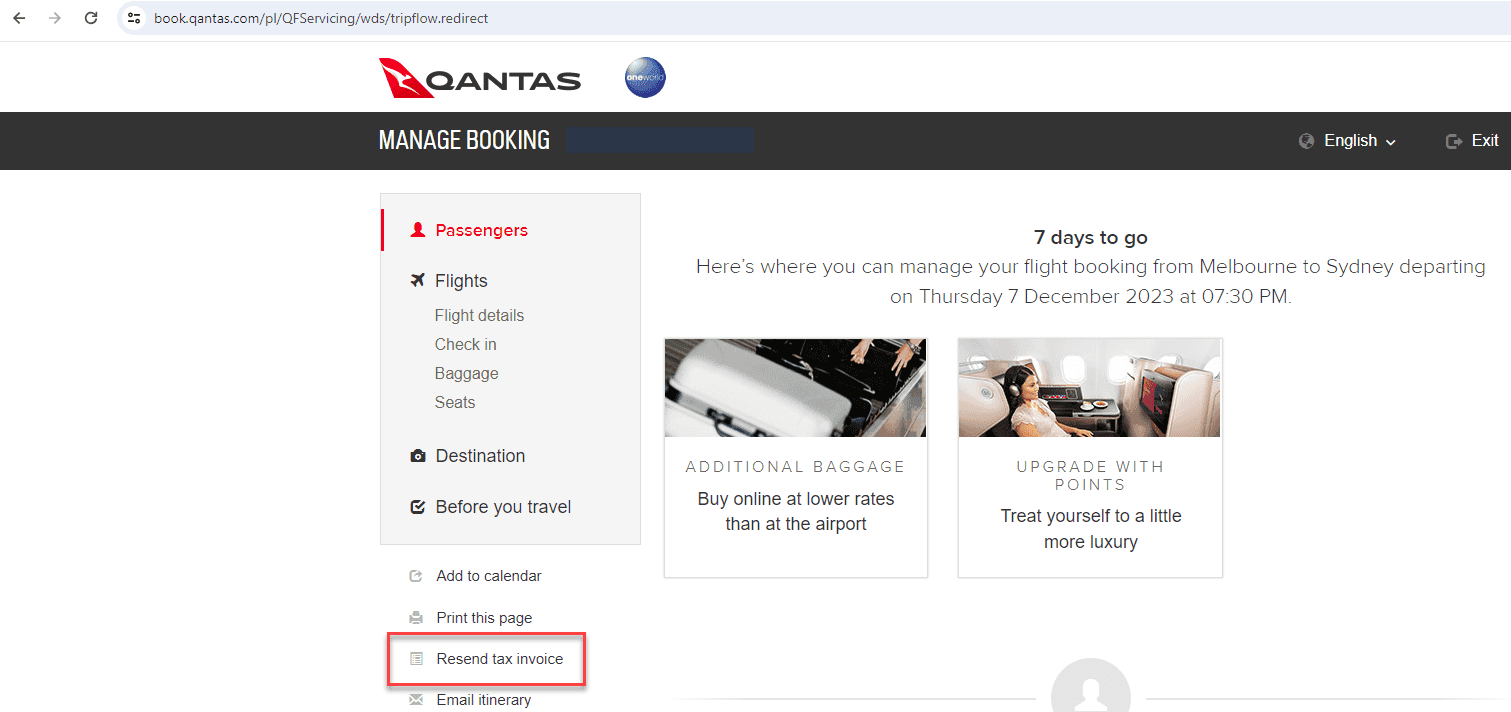The image is a screenshot from the Qantas website, specifically the "Manage Booking" section. The URL displayed in the address bar reads "book.qantas.com/pl/QF_servicing/B_noWDS/trip_float_redirect." At the top of the page, the Qantas logo is prominently displayed, followed by a black navigation bar featuring options such as "Manage Bookings." On the right side of this bar, there is a language selection drop-down menu currently set to "English."

Below this navigation bar, the page lists various options available under "Manage Booking." These include: "Passengers," "Flights," "Flight Details," "Check-in," "Baggage," "Seats," "Destination," "For You," and "Travel." Directly below these options, users are offered additional actions: "Add to Calendar," "Print this Page," "Resend Tax Invoice," and "Email Itinerary." Notably, the "Resend Tax Invoice" option is highlighted with a red box, indicating its importance or recent selection.

The central part of the page contains a message informing the user that there are "7 days to go" until their flight, providing an option to manage their booking for a flight from Melbourne to Sydney. The flight is scheduled to depart on Thursday, December 23rd, at 7:30 PM.

Additional services are promoted below this notification, such as "Additional Baggage: Buy Online at Lower Rates than at the Airport," and "Upgrade with Points: Treat Yourself to a Little More Luxury."

At the bottom of the page, there is a grey line featuring a small person icon in the center, adding to the clean and professional layout of the website. Overall, the highlighted "Resend Tax Invoice" option suggests the user may be focused on financial documentation for their trip.